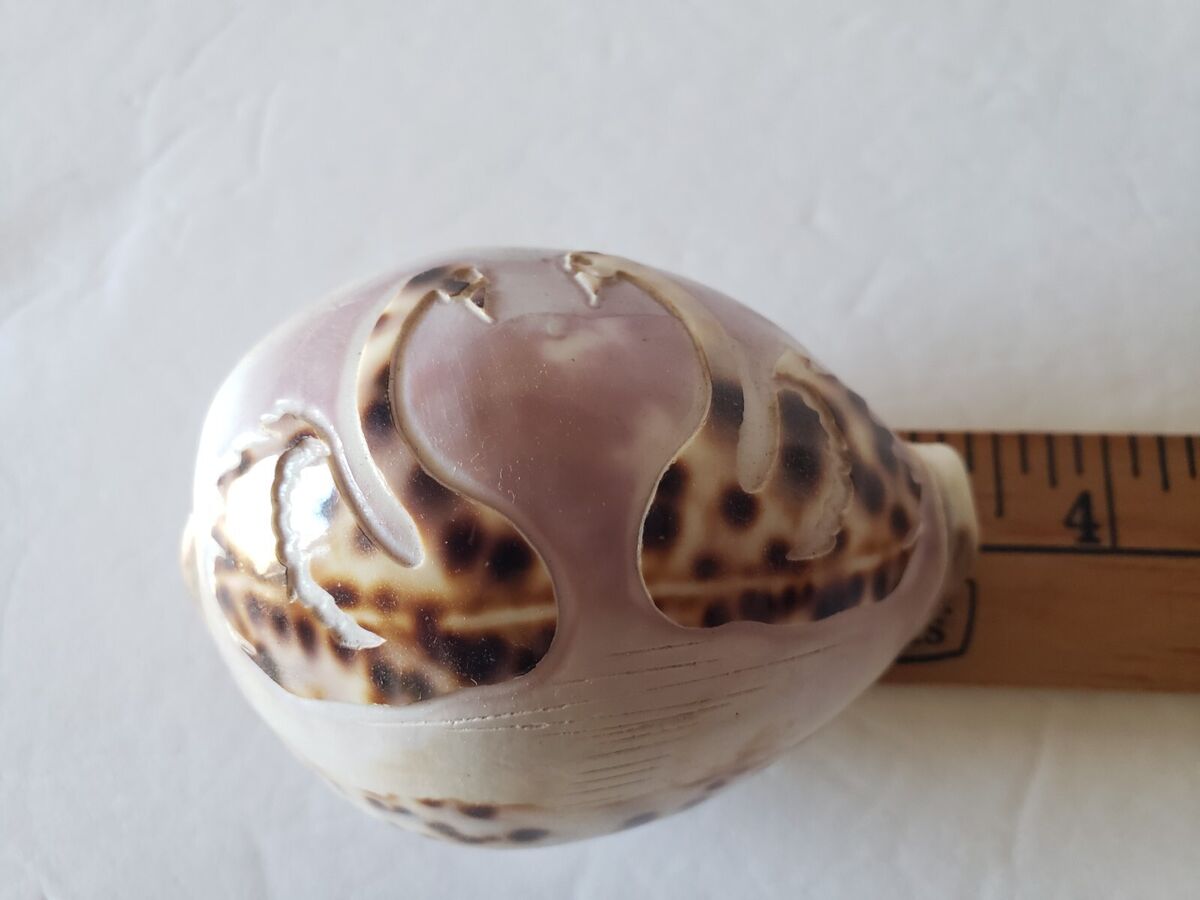This close-up photograph showcases a meticulously carved seashell centered on a wooden ruler, which measures the shell to be just under four inches in width. The shell's exterior is artistically transformed into a detailed depiction of two swans, their elegant heads meeting to form a heart shape. The swans' interiors feature a blend of black, white, and light brown hues, while the shell's outer surface displays shades of white and light purple. The image, captured with a focus on the intricate craftsmanship, has the shell positioned slightly towards the bottom of the frame, with the ruler placed vertically to its right, numbered to indicate the shell's size. The photograph likely taken indoors, highlights both the artistry involved in the carving and the detailed texture of the seashell.